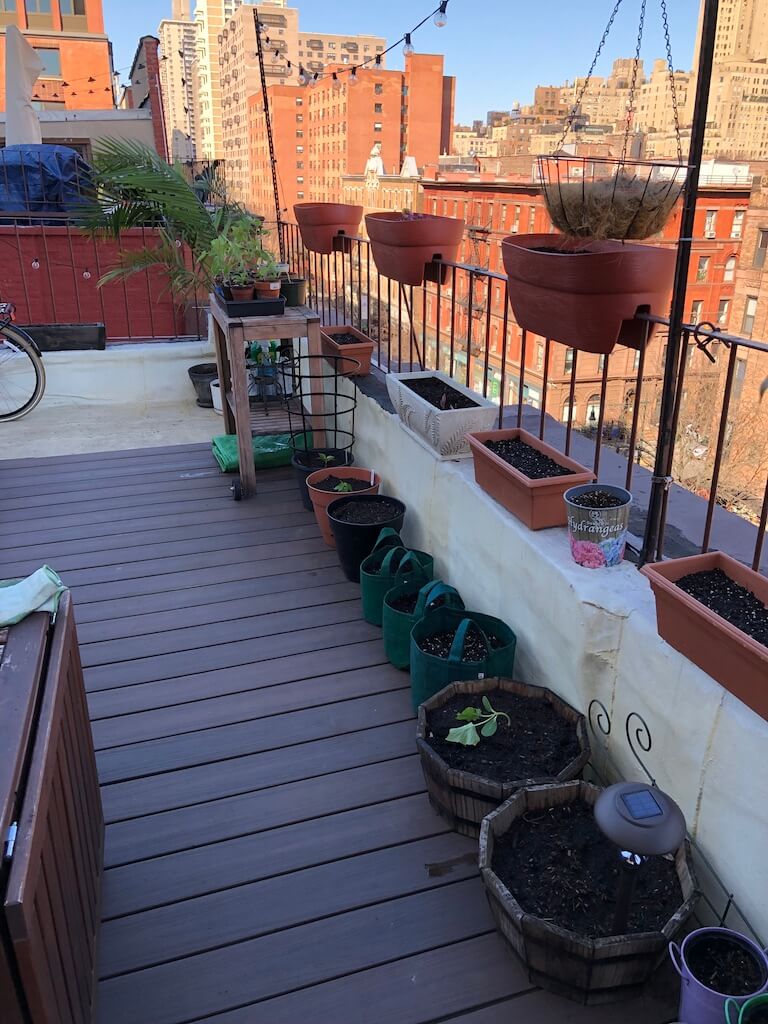The photograph captures a vertically aligned, rectangular patio terrace on the rooftop of a tall building in a city, with multiple multi-story red brick buildings visible across the street. The terrace is covered with dark brown wooden planks and contains an array of gardening elements and furniture. On the left side of the image, a brown outdoor chest is topped with silver hinges and white and green gardening gloves. A low white wall to the right features a black metal railing adorned with numerous potted plants, including terracotta pots and hanging baskets. Many of the pots appear to contain soil, with a few showing the beginnings of green leaves. The wooden flooring hosts additional potted plants and a small brown table, further back, also bearing potted plants. In the left portion of the image, part of a bicycle tire is visible, and in the background, the cityscape of brown and tan buildings stretches under a blue sky.